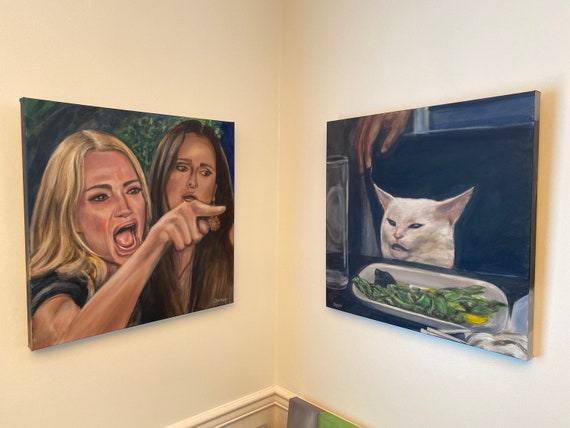This photograph captures an art exhibit featuring two detailed oil paintings inspired by the famous meme involving a woman yelling at a bemused white cat. The paintings are mounted on adjacent sides of a light beige corner wall. 

On the left, the painting depicts the blonde woman from the meme, wearing a black shirt and pointing her finger accusatorily. Behind her stands a brunette woman attempting to calm her. The background is a mix of green and blue hues, with a tree visible behind the blonde woman.

On the right, the second painting shows the white cat with a mischievous expression, sitting in front of a plate of food that appears to contain greens and a slice of lemon. An empty glass is placed to the left of the cat, and the background features blue tones.

Together, these hand-painted canvases capture the humor and iconic imagery of the meme, showcasing the artistic transformation of a digital moment into classic oil paintings.